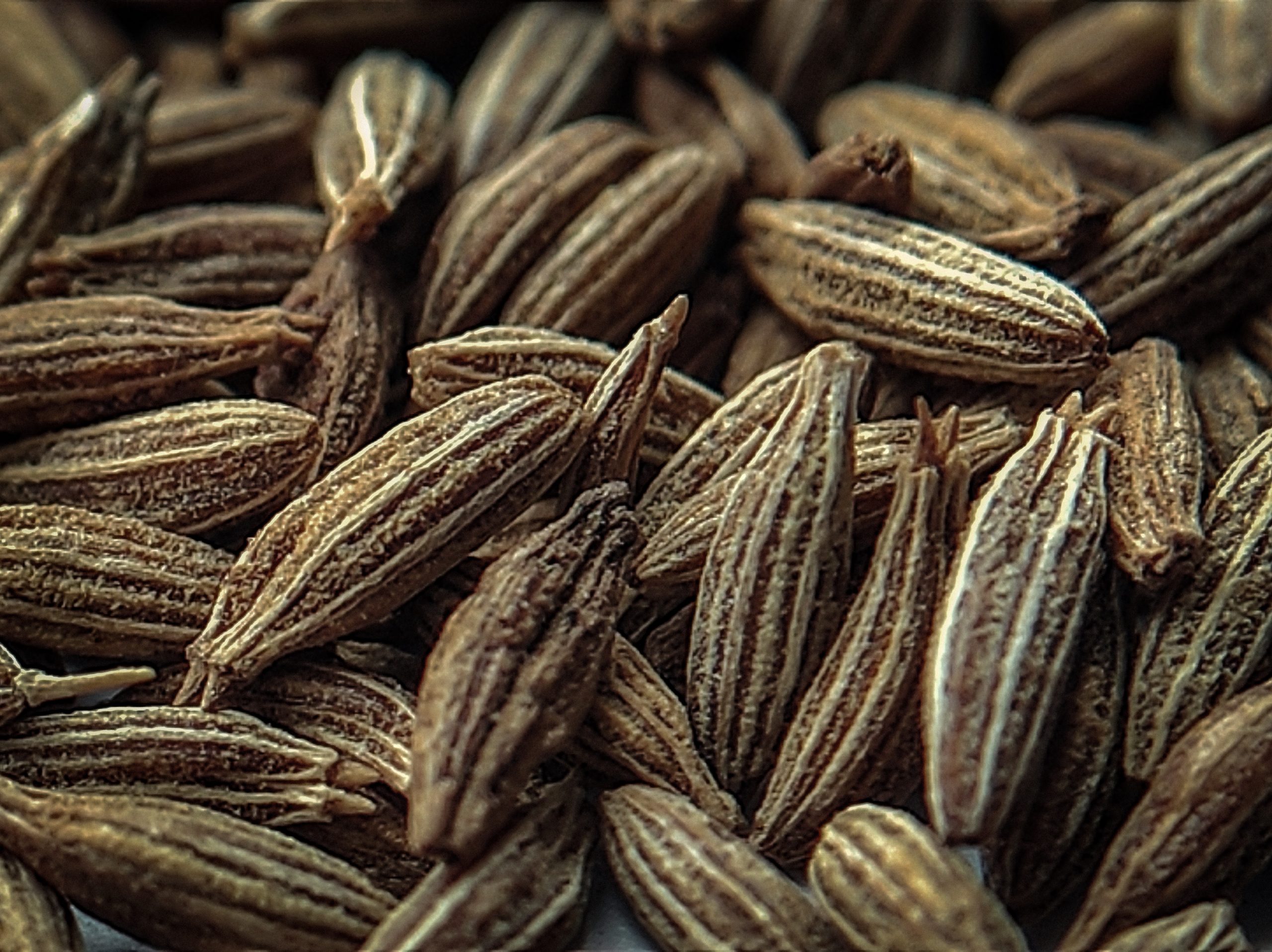The image depicts a detailed close-up of an extensive pile of brown seed pods, resembling elongated ovals or narrow footballs. Each pod is predominantly brown with tan vertical stripes running along its length, providing a distinct textured appearance. The pile spans the entire frame from bottom to top and left to right, with no visible background elements. Some pods are in sharp focus while others in the background are blurred, highlighting the depth and density of the pile. The pods vary in size and orientation—some are horizontal, some vertical, and some diagonal. There are at least 30 to 50 pods visible, each appearing hard and possibly about a centimeter or less in length. The exact type of seed pod is unclear, though they are likely intended for planting or growing purposes.